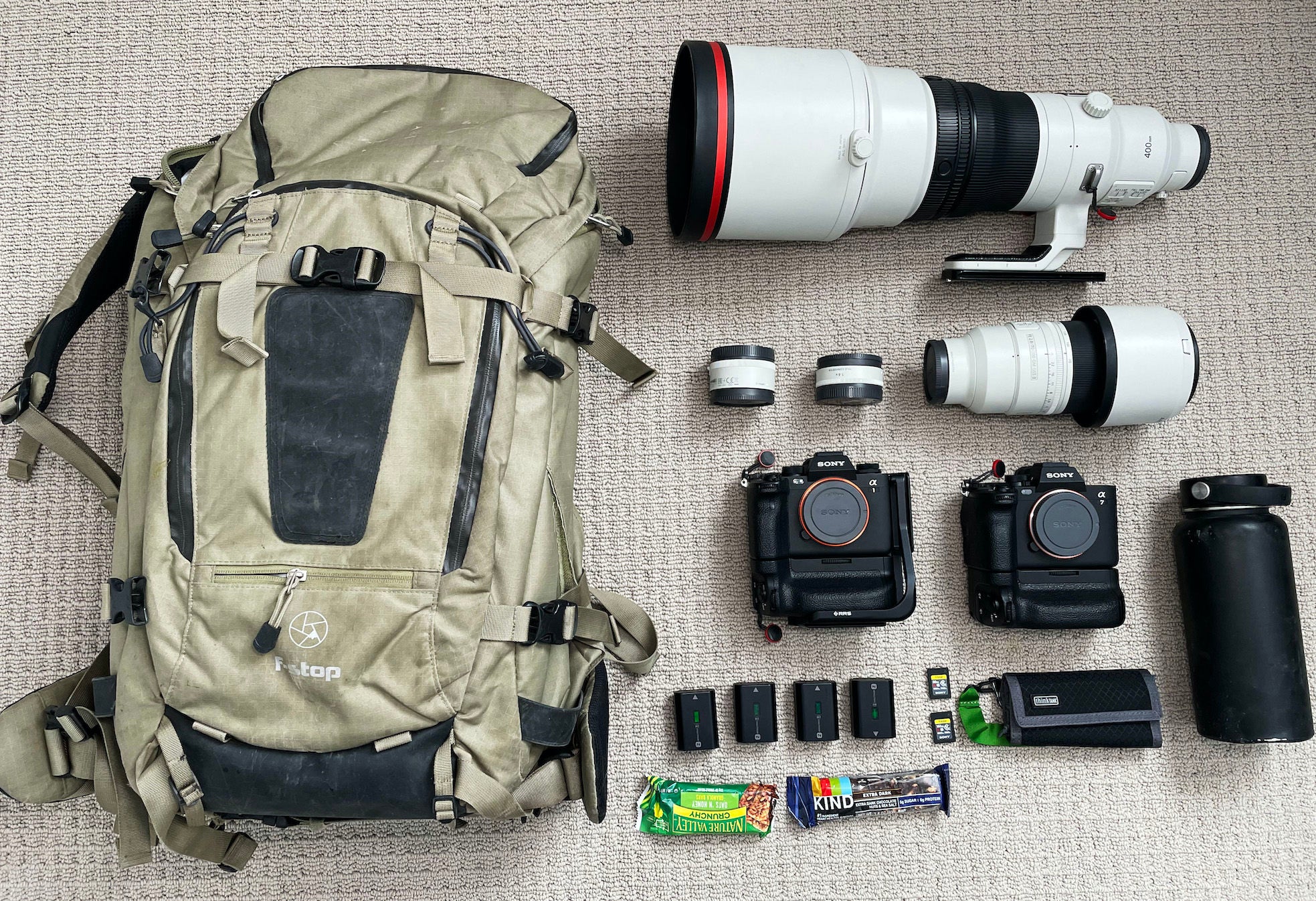On a beige carpet, a meticulously arranged collection of a greenish-tan backpack and photography gear is laid out. The backpack, marked with the F-Stop brand in white text and featuring a camera shutter logo, dominates the left side of the image with its numerous black-accented straps, buckles, and zippers. To its right, there are two Sony cameras, a gigantic camera lens, a smaller lens, and additional smaller lens attachments, likely lens filters. Accompanying these are various black objects, plausibly batteries and memory cards essential to the camera equipment. A black water bottle rests nearby. At the bottom of the layout, an upside-down Nature Valley crunchy bar and a Kind bar complement the setup, hinting at preparedness for a day of photography, possibly combined with hiking. The overall scene is suggestive of a well-equipped photographer's backpack, ready for an outdoor adventure.